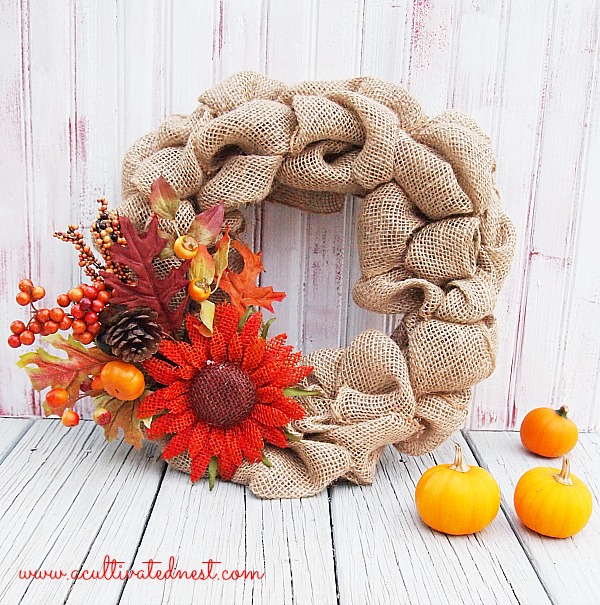This professional product photo showcases a beautifully crafted autumnal wreath made from burlap. The image, with a square format, features the wreath prominently displayed against a whitewashed beadboard wall, resting on weathered wood planks, possibly a picnic table or deck flooring. The wreath itself is elegantly adorned on the bottom left with artificial red oak leaves, red silk flowers, artificial berries, and mini gourd or pumpkin shapes. A real pine cone and a large sunflower, made of burlap with orange petals and a brown center, add charming touches to the design. Additionally, there are three small miniature pumpkins positioned to the right of the wreath; one appears natural, while the other two have stems painted in gold. The overall aesthetic embodies the essence of autumn with warm, earthy tones and a rustic feel. A red script watermark reading "www.occultivatednest.com" is displayed at the bottom left corner of the photo, hinting at a home decor website.